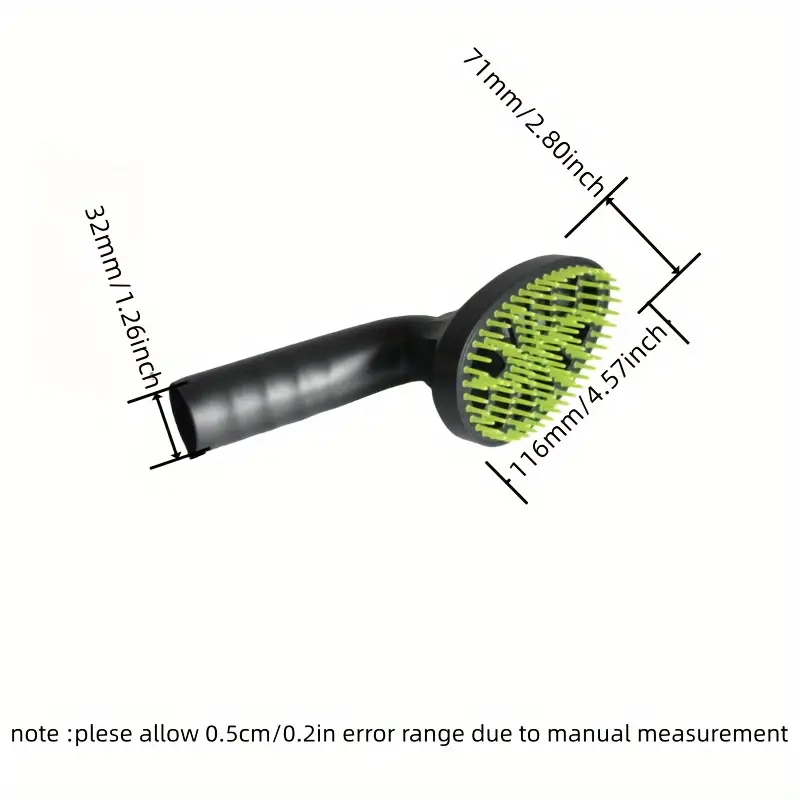The image depicts a digital art illustration of a black brush attachment with a rubber handle and yellow spikes, commonly used for cleaning or grooming purposes. The brush is centrally positioned against a white background. Detailed measurements are displayed around the brush: the bottom opening measures 32 millimeters (1.26 inches), the width of the head is 71 millimeters (2.8 inches), and the height of the head is 116 millimeters (4.57 inches). A note at the bottom of the image, albeit with a typographical error ("please" spelled as "plese"), advises viewers to allow a 0.5 centimeter (0.2 inch) margin of error due to manual measurement. The overall presentation suggests that this image could be from an online retail listing, offering precise dimensions for potential buyers.